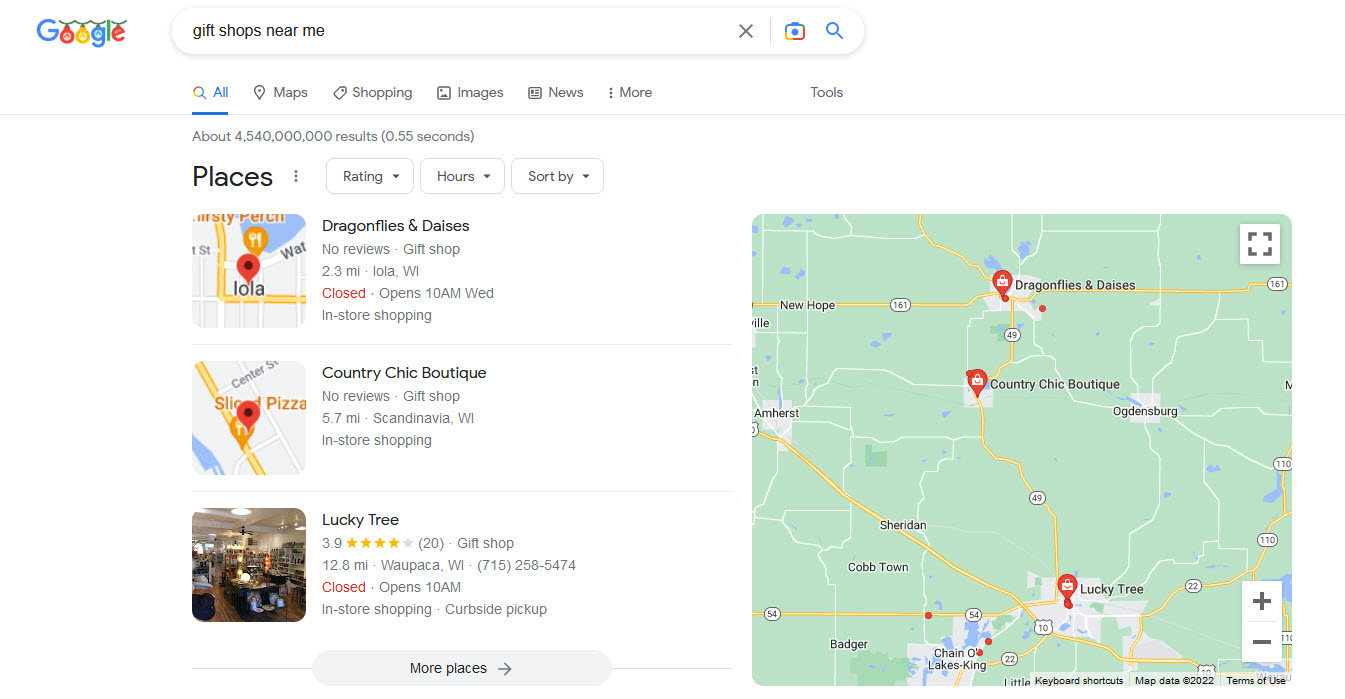The image depicts a Google search results page for the query "gift shop near me." On the left side of the search bar, the Google logo is decorated to resemble Christmas ornaments. The search yielded approximately 4.54 billion results in 0.55 seconds.

Below the search bar, navigation options include: All, Maps, Shopping, Images, News, More, and Tools. The results provide information such as places, ratings, hours of operation, and sorting options. 

The first result is for "Dragonflies and Davies," a gift shop located 2.3 miles away in Iola, Wisconsin. Currently, it has no reviews and is closed but will open at 10 a.m. on Wednesday, offering in-store shopping.

The second result is for "Country Chick Boutique," another gift shop, situated 5.7 miles away in Scandinavia, Wisconsin. It also has no reviews and offers in-store shopping.

The third result is for "Lucky Tree," a gift shop with a rating of 3.9 stars based on 20 reviews. It is located 12.8 miles away in Waupaka, Wisconsin. The contact number provided for Lucky Tree is 715-258-5474.